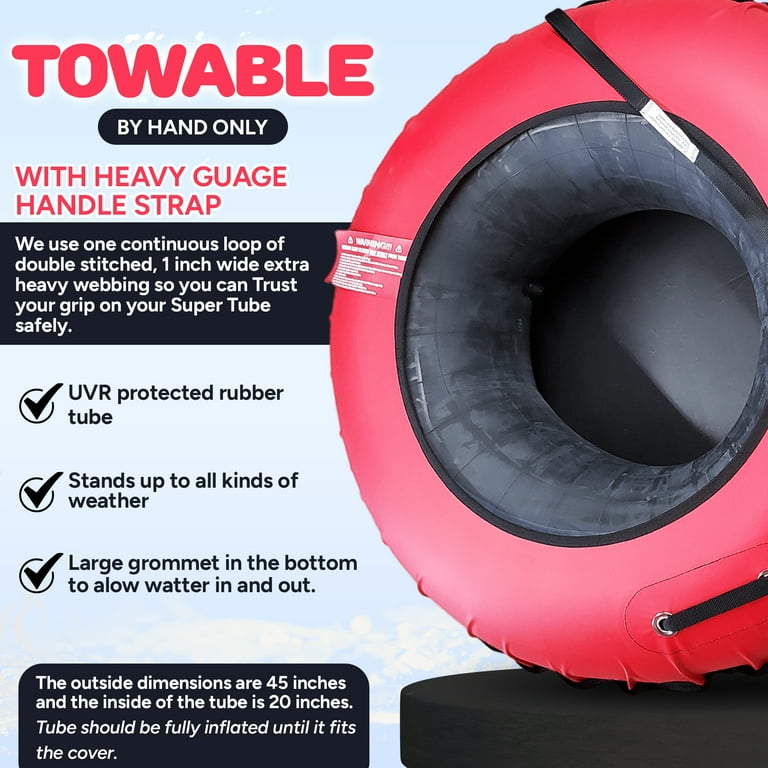This detailed advertisement showcases a vibrant circular tube prominently positioned on the right side of the image, standing vertically on a black surface. The tube features a striking color combination with a red outer rim and an inner black circle, accentuated by black straps for easy handling. The left side of the poster is dominated by text in red and white, set against a contrasting blue background. The ad highlights key product features with a checklist of three items at the center-left: "UVR Protected Rubber Tube," "Stands up to all kinds of weather," and "Large grommet in the bottom to allow water in and out." The main headline at the top reads, "Towable by Hand Only with Heavy Gauge Handle Strap," emphasizing the durable design. The accompanying text elaborates: "We use one continuous loop of double-stitched, one-inch wide heavy webbing so you can trust your grip on your super tube safely." At the bottom, detailed specifications inform that the tube's outside dimensions are 45 inches, with an inside diameter of 20 inches, and it should be fully inflated to fit its cover.